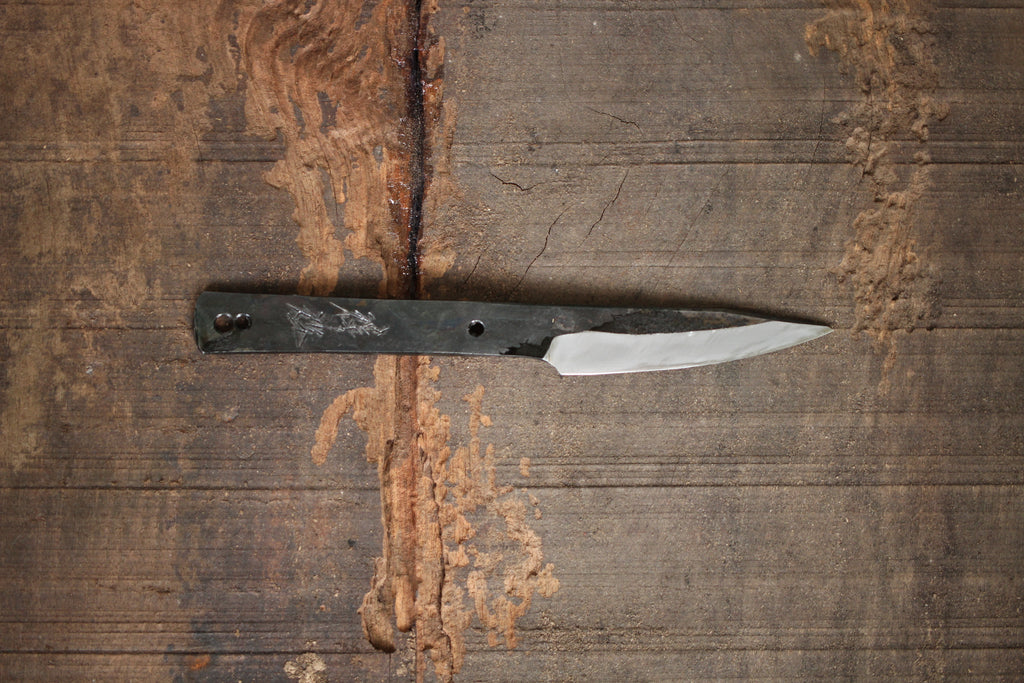This photograph features a close-up, precisely centered top-down view of a knife resting on a distressed, grayish-brown wooden surface. The background, which could be an old table, counter, or floor, showcases prominent horizontal lines that give it a wood-like appearance, though it might also be concrete mimicking wood grain. The surface is heavily weathered, with areas where the top layer has peeled off, revealing brown and yellowish streaks, and there are deep, gouged lines running across it, suggesting significant wear and tear or intentional carving.

The knife itself is oriented with its blade pointing to the right. The blade is silver at the bottom of the image, transitioning to a dark charcoal grayish-black towards the top. The handle is a bare metal, also in a charcoal grayish-black hue, featuring several holes near the end, possibly for hanging or attaching purposes. The craftsmanship of the knife appears utilitarian, with a sharp blade that shows signs of chipping, revealing blackish spots where the surface material has worn away. Debris from the heavily scored surface is scattered around, enhancing the rugged and beaten-up appearance of both the knife and the background.